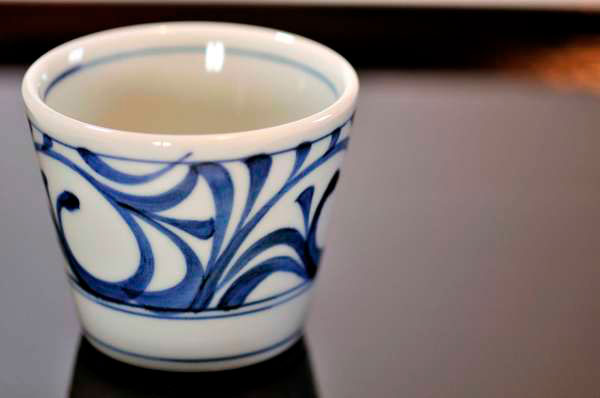This full-color square photograph, taken indoors with artificial lighting, artistically showcases a white ceramic teacup without a handle, suggesting it could also be described as a porcelain cup. The focal point is the intricately decorated cup, which features a series of horizontal blue lines around its exterior, sandwiching a detailed pattern of swirly blue leaves or vines. The inside rim of the cup also displays a blue trim. The cup itself sits prominently against a dark, out-of-focus tabletop, likely wood, that provides a rich contrast to its gleaming white surface. The composition is minimalistic with no border framing the image, allowing the viewer to focus solely on the beautifully detailed cup. The photo captures the cup casting a subtle shadow, hinting at its three-dimensional form, and draws attention to its clean lines and decorative details.